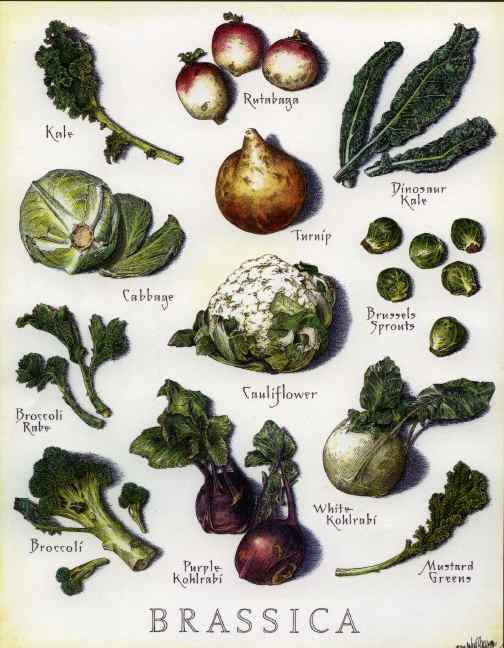This image, resembling a vintage-style poster one might find in a rustic kitchen or restaurant, showcases a variety of root vegetables all belonging to the Brassica family. The poster is framed with a brownish edge, giving it an aged appearance. Along the bottom, the word "Brassica" is elegantly displayed. Each vegetable is depicted with its name beside it in a sophisticated font. Among the illustrated vegetables, you see kale, rutabaga—depicted as round with red tops and white bottoms—alongside green-hued dinosaur kale. Other included Brassica family members are cabbage, turnip, Brussels sprouts, multiple varieties of kohlrabi (purple and white), broccoli, broccoli rabe, cauliflower, and mustard greens. Most of these vegetables are green or cruciferous, prominently representing the Brassica family’s diversity in the image, which, despite its low resolution, details each plant type distinctly.